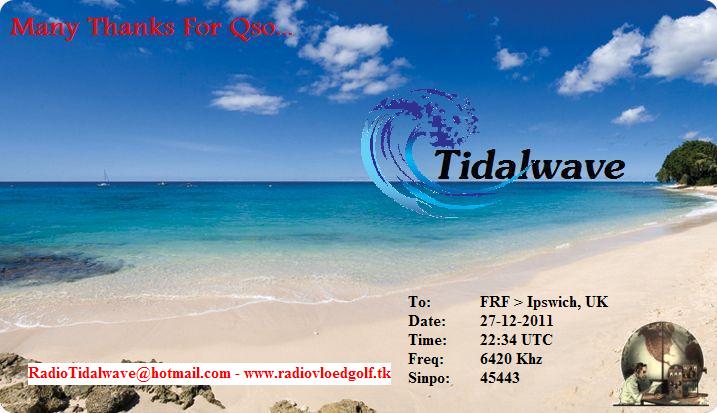This image appears to be a nostalgic, digitally-compressed advertisement or announcement, possibly for a radio event or QSO (communication between amateur radio operators), set against a scenic beach backdrop. The photograph showcases a serene ocean with a sandy beach on the right, a clear blue sky adorned with a few wispy clouds, and several sailboats visible in the corner, evoking a tranquil seaside setting.

Overlaying the photo, in the top left corner, the text reads, "Many Thanks for a QSO." Toward the right center of the image, there is a poorly rendered clipart graphic of a wave next to the words "Tidal Wave," with remnants of a white background still visible, suggesting the clipart was not properly cut out. 

At the bottom, enclosed within a white rectangular border, the text provides detailed event information: "RadioTidalWave at Hotmail.com - www.radioVLOEDGulf.tk, 2FRF Ipswich, UK, date 27-12-2011, time 22:34 UTC, frequency 6420 kHz, SYNPOL 45443." Additionally, the bottom right corner features an illustration of an old radio operator in front of a globe.

The color scheme of the advertisement comprises beige, blue, aqua blue, white, dark blue, dark green, gray, black, red, and brown, contributing to the overall vintage feel of the image.